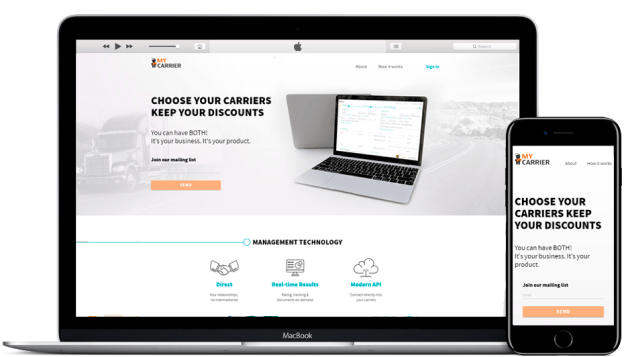The promotional image showcases two Apple devices, a MacBook on the left and an iPhone on the right, both displaying a similar webpage or application interface. The MacBook, distinguishable by its silver keyboard and curved edges, features a detailed display within the iTunes app. Visible elements on the screen include playback controls and a volume adjustment button at the top, along with prominent text reading, "My career, choose your carriers, keep your discounts. You can have both, it’s your business, it’s your product." Additionally, there is a call to action to join a mailing list, with a text box for entering an email address and an orange submission button.

Further down on the MacBook's screen, the content continues with the heading "Management Technology," accompanied by graphic images: one of two hands clasping, another of a computer screen line drawing, and a cloud icon with the text "API" beneath it.

The iPhone, a model released before the iPhone X era identifiable by its circular home button for fingerprint unlocking, displays a simplified version of the same webpage. It retains the key phrase "choose your carriers, keep your discounts. You can have both," but omits the fuller textual and graphical content visible on the MacBook’s larger screen. This image effectively underscores the synergy and integrated interface between different Apple devices for accessing the same web services or applications.